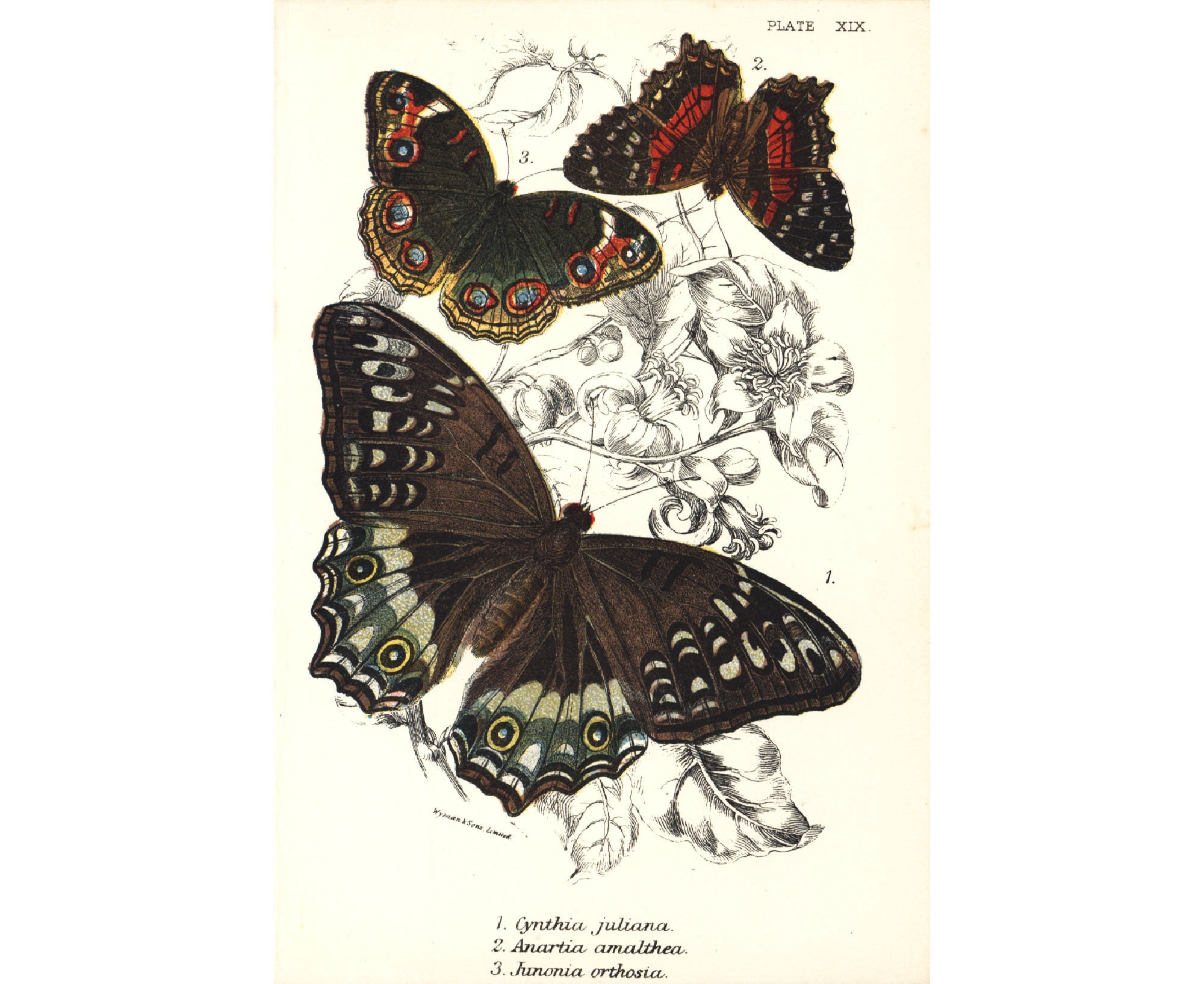In this beautifully detailed illustration labeled "Plate 19," we observe three butterflies of distinct and striking designs set against a pristine white background. The uppermost butterfly, marked as Number 2, hangs upside down and showcases a splendid combination of red, black, and white hues. Its intricate patterning draws the viewer's eye with its vibrant contrast. Below it, the second butterfly displays wings adorned with a blue, jewel-like, twirly pattern, accented with touches of red and gold, lending it an almost regal appearance. The most prominent of the trio, positioned at the bottom, features elegant shades of gray, ranging from light to dark, punctuated by distinctive circular markings with black dots at their centers. Interspersed among these butterflies are delicate drawings of leaves and flowers, adding a botanical element to the composition. Beneath the illustration, there is additional writing which provides context or further details about the depicted scene.